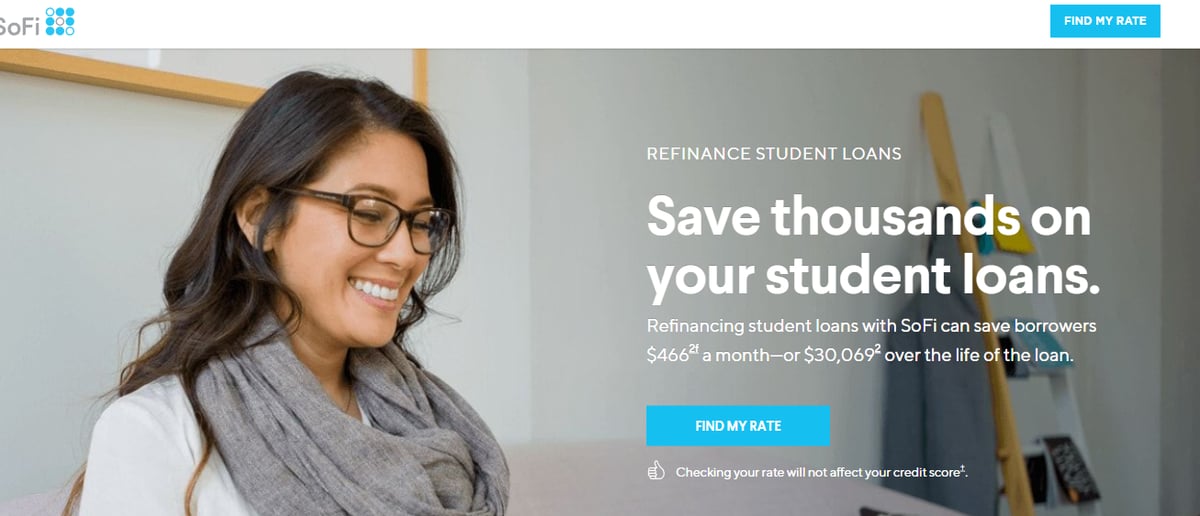This image from the SoFi website features several design elements and text aimed at promoting their loan refinancing services, specifically for student loans. The SoFi emblem, comprised of blue and white circles, is prominently displayed to the right. 

Central to the promotional message is the "Find My Rate" button, urging users to check their current rates without affecting their credit score, as indicated by the thumbs-up icon next to this assurance. 

The headline, stating "Save thousands on your student loans," is written in bold white text, highlighting the benefits of refinancing with SoFi. Further details below inform borrowers that they can save an average of $466 monthly, totaling approximately $30,000 over the life of a loan. 

The image features a smiling woman, likely of Asian descent, who exudes a friendly, approachable air. She is wearing a gray scarf, has medium to long black hair, glasses, and is standing in what appears to be a classroom, as indicated by the chalkboard behind her. Surrounding her are various items, including a coat rack holding jackets and possibly an iPad, suggesting a well-organized, professional environment.

Overall, this image and accompanying text effectively communicate the financial advantages of SoFi's loan refinancing services in a warm, inviting context.